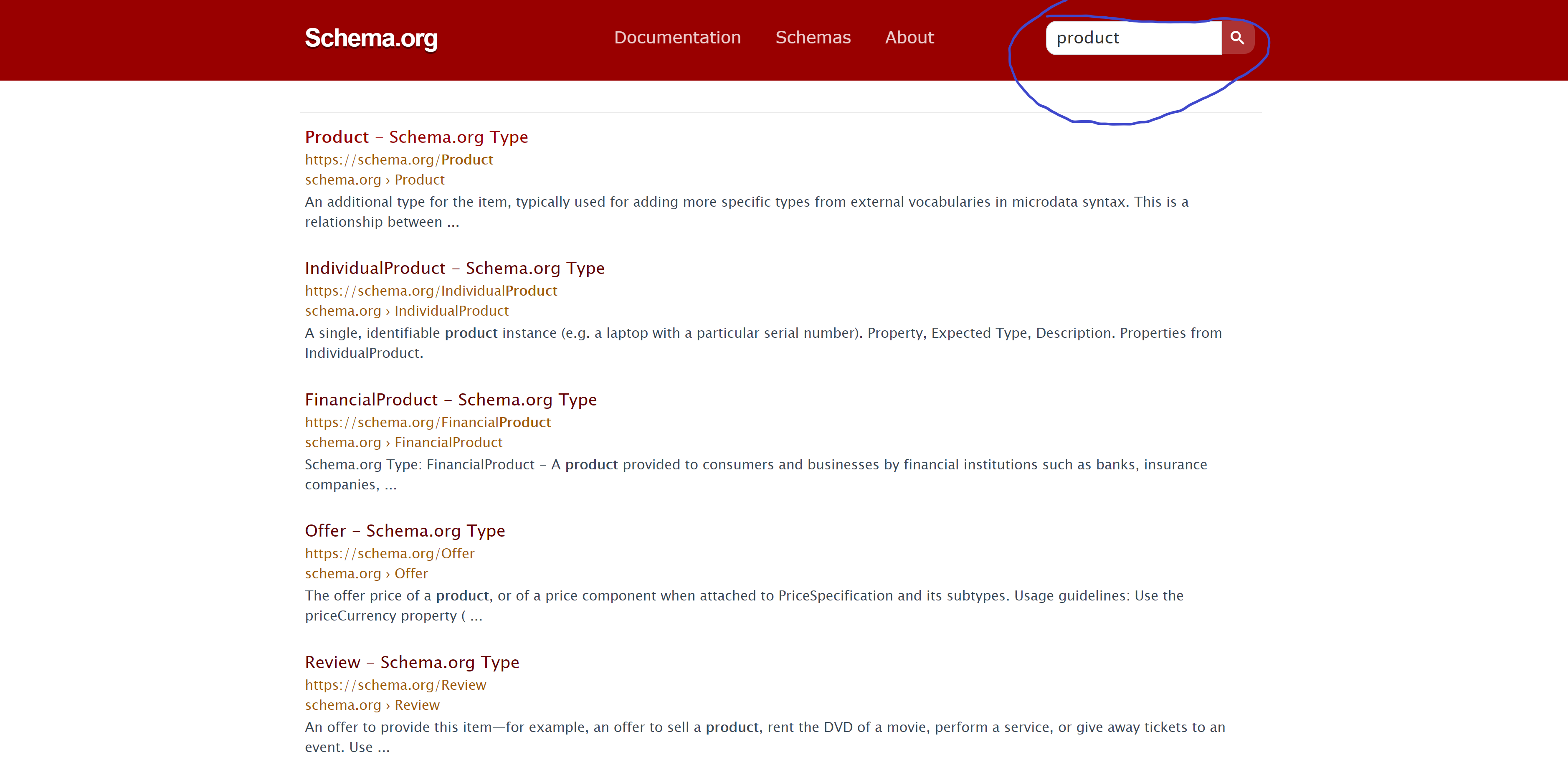In the image, the top section features a red background with the text "schema.org" on the left-hand side in white. Just below, there's a white text that reads "documentation," which appears to be related to "Schemas About." Positioned centrally is a white search bar, which ends with a red button featuring a white magnifying glass icon; this button is circled in blue.

Directly underneath, the text "product schema.org type" is displayed in red. Below this, in orange, it shows the URL "https://schema.org/Product." An arrow points from "schema.org" to "Product" indicating a relationship. The explanatory text in black states: "Additional type for the item typically used for adding more specific types from external vocabularies in microdata syntax. This is a relationship between..."

Next, the text "Individual product - schema.org type" is highlighted in red. The following URL, "https://schema.org/IndividualProduct," appears in orange. A detailed description in black provides further clarity: "A single identified product instance (e.g., a laptop with a particular serial number). Property expected type: Description of properties from IndividualProduct."

Additionally, three other schema types are listed in sequence:
- "Financial product schema type" in red,
- "Offer schema type" in red,
- "Review schema type" in red.

Each of these is followed by the associated URLs in orange:
- "https://schema.org/FinancialProduct,"
- "https://schema.org/Offer,"
- "https://schema.org/Review."

Each URL is accompanied by the corresponding schema.org type mentioned: "Financial Product," "Offer," and "Review."